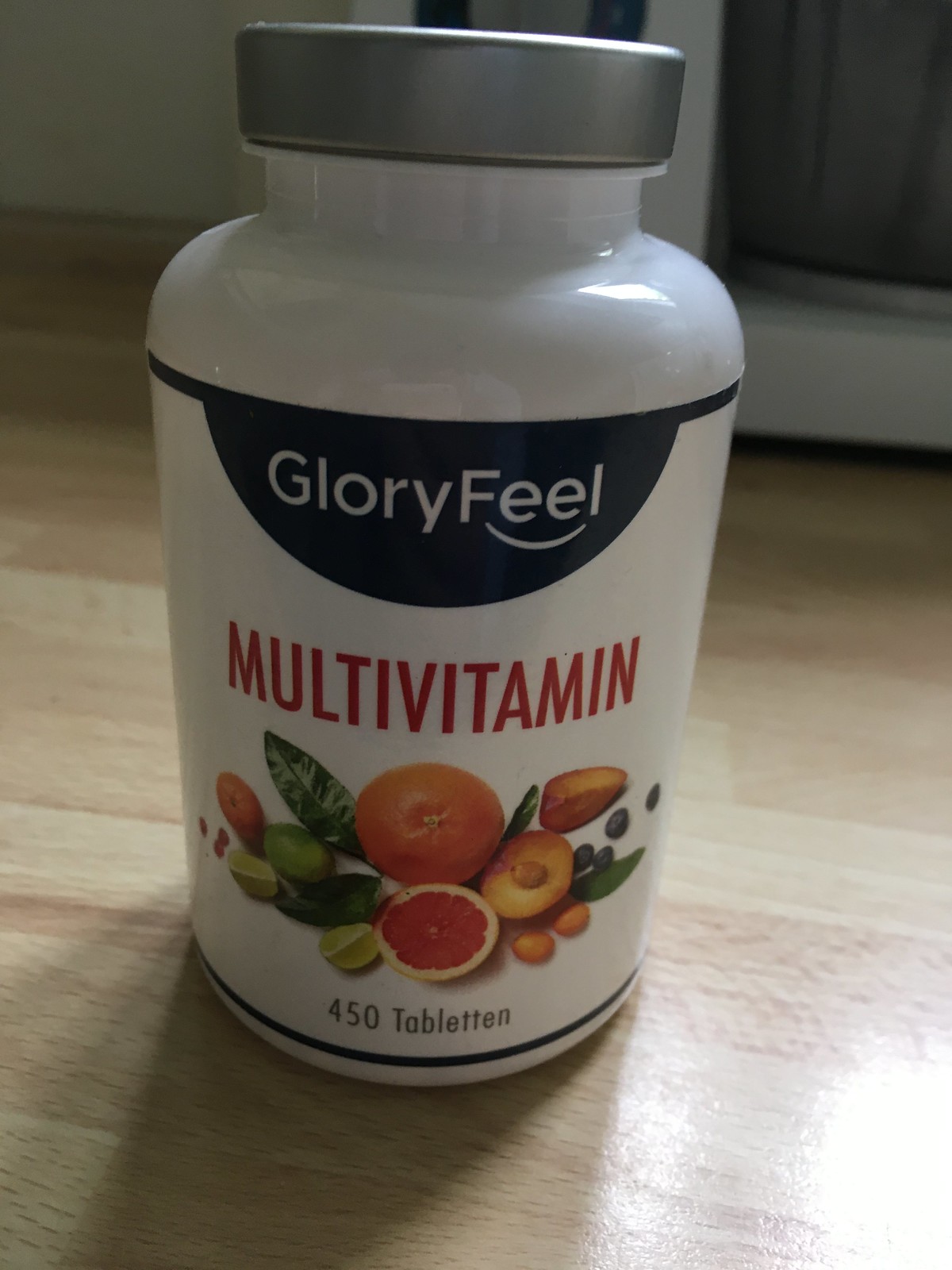This is an indoor close-up photo of a white bottle of multivitamins, likely resting on a light brown or beige table or floor. The bottle features the brand name "GLORY FEEL" in white lettering against a dark blue background at the top, with a design incorporating a smile under the E's of "FEEL" to create eyes. It tapers up to a gray cap. Below the brand name, in red text, it reads "multivitamin." The lower part of the bottle showcases illustrations of various fruits, including an orange, lemon, lime, blueberries, possibly some grapes, and an avocado half, along with some leaves. Beneath these images, in what appears to be black text, it is labeled "50 tableten," which suggests "50 tablets" in another language.